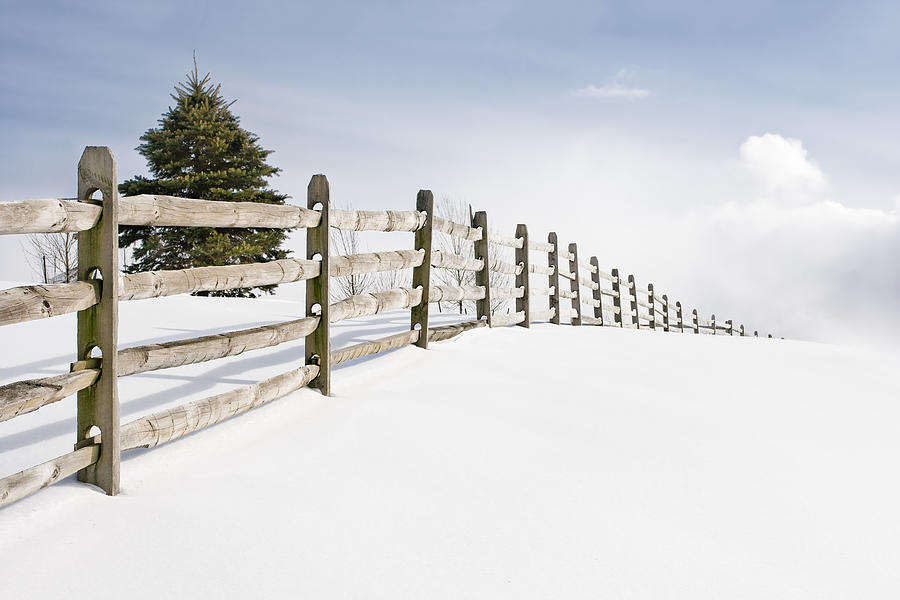The image depicts a serene, snow-covered field under a partly cloudy daytime sky with patches of blue peeking through. Dominating the scene is a weathered wooden fence that starts about 20% up from the left side of the image, consisting of four horizontal beams and posts that stretch into the distance, gradually diminishing in height as it follows a winding path, initially moving right and then undulating over a gently rising hill. The immaculate, untrodden snow blankets the entire field, lending an untouched and tranquil feel to the landscape. To the left of the fence stands a tall, verdant pine tree, likely a couple of stories high, adding a splash of green to the predominantly white scene. Further left, among the bare-branched trees, the fence creates a natural boundary that leads the eye into the horizon. This peaceful winter day is beautifully captured with the soft light and fluffy clouds in the sky.